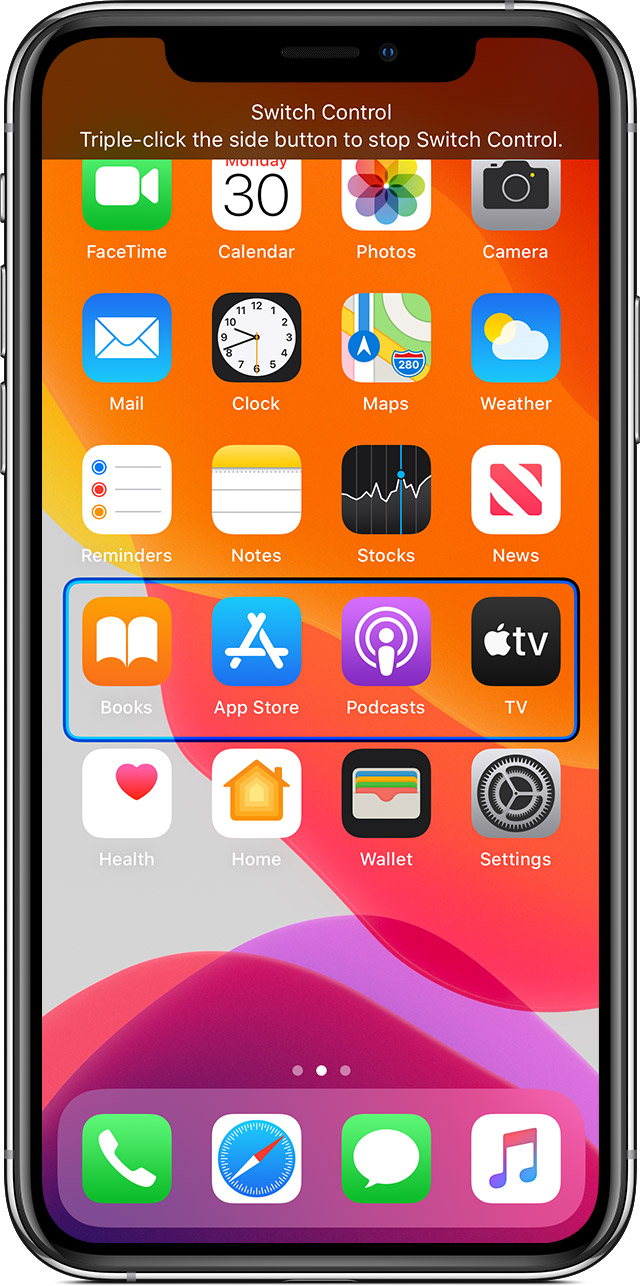This image features a vertically-oriented smartphone screen displaying the main home screen interface with various app icons. At the top of the screen, there's a narrow, horizontal, brownish section with white text that reads "Switch Control." Below this, in smaller white text, it instructs, "Triple-click the side button to stop Switch Control."

The home screen is organized into several rows of app icons, each vividly depicted:

1. **First Row:**
   - A green rectangle with a white camera icon labeled **FaceTime**.
   - A white calendar icon with the number "30" and the label **Calendar**.
   - A white rectangular icon with multicolored petals, labeled **Photos**.
   - A gray icon with a black camera, labeled **Camera**.

2. **Second Row:**
   - A blue-to-turquoise gradient background with a white envelope, labeled **Mail**.
   - A clock icon with the label **Clock**.
   - A map icon labeled **Maps**.
   - A weather icon depicting a blue sky, sun, and cloud, labeled **Weather**.

3. **Third Row:**
   - A white background with horizontal lines and bullet points, labeled **Reminders**.
   - A yellow notepad icon labeled **Notes**.
   - A black and white graph icon labeled **Stocks**.
   - A white background with an "N" logo, labeled **News**.

4. **Fourth Row:** Enclosed in a blue rectangle.
   - An orange background with an open book icon, labeled **Books**.
   - A turquoise background with a white "A" icon, labeled **App Store**.
   - A purple background with a white microphone, labeled **Podcasts**.
   - A black icon with a white Apple logo and "TV" labeled **TV**.

5. **Fifth Row:** Not enclosed in the blue rectangle.
   - A white background with a red heart, labeled **Health**.
   - A white background with a yellow-orange house, labeled **Home**.
   - A black icon with a white wallet, labeled **Wallet**.
   - A gray icon with gears, labeled **Settings**.

6. **Sixth Row:**
   - A green background with a white telephone icon (no label).
   - A white icon with a compass (no label).
   - A green icon with a white speech bubble (no label).
   - A white background with black musical notes (no label).

This comprehensive view of the smartphone's home screen provides detailed visual and textual descriptions of each app icon and their respective locations.